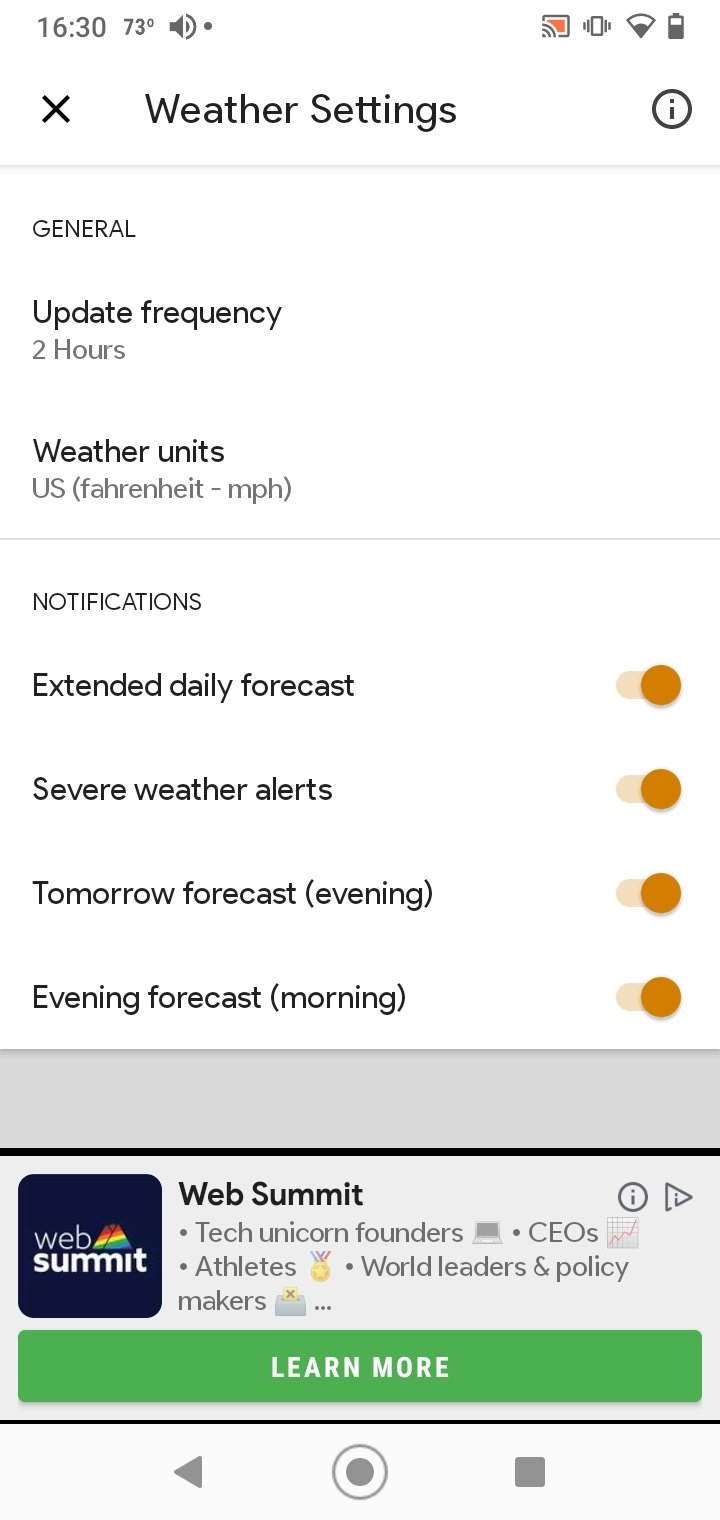This image is a detailed screenshot of a smartphone displaying the "Weather Settings" section within a weather application. The interface has a clean, white background. At the very top, the screen shows the current time, 16:30, and the temperature, 73 degrees Fahrenheit. The battery icon in the upper right corner appears nearly full, indicative of a well-charged phone.

The header of this settings screen reads "Weather Settings," flanked by an 'X' on the left for closing the settings and a circular icon with a lowercase 'i' on the right, likely for informational purposes. Immediately below this header is a divider line.

The topmost section under the header features a white rectangle labeled "General". Beneath this, "Update Frequency" is mentioned with the interval set to "2 hours." Moving further down, the next heading is "Weather Units," which shows the units as "US Fahrenheit (mph)".

Another divider line separates the "General" section from the following "Notifications" section, which contains four items:
1. "Extended Daily Forecast" with an orange toggle switch turned on.
2. "Severe Weather Alerts," also toggled on.
3. "Tomorrow Forecast (Evening)," toggled on.
4. "Evening Forecast (Morning)," toggled on.

At the very bottom of the screen, there is a gray area labeled "Web Summit." To its right, a blue box also labeled "Web Summit" features a rainbow-colored tent icon. The accompanying text highlights the event's significance by mentioning "Tech unicorn founders, CEOs, athletes, world leaders, and policymakers." Below this promotional content, a green button labeled "Learn More" is available for further information.

Overall, the image provides a comprehensive look at various weather settings and a promotional banner for an upcoming event.